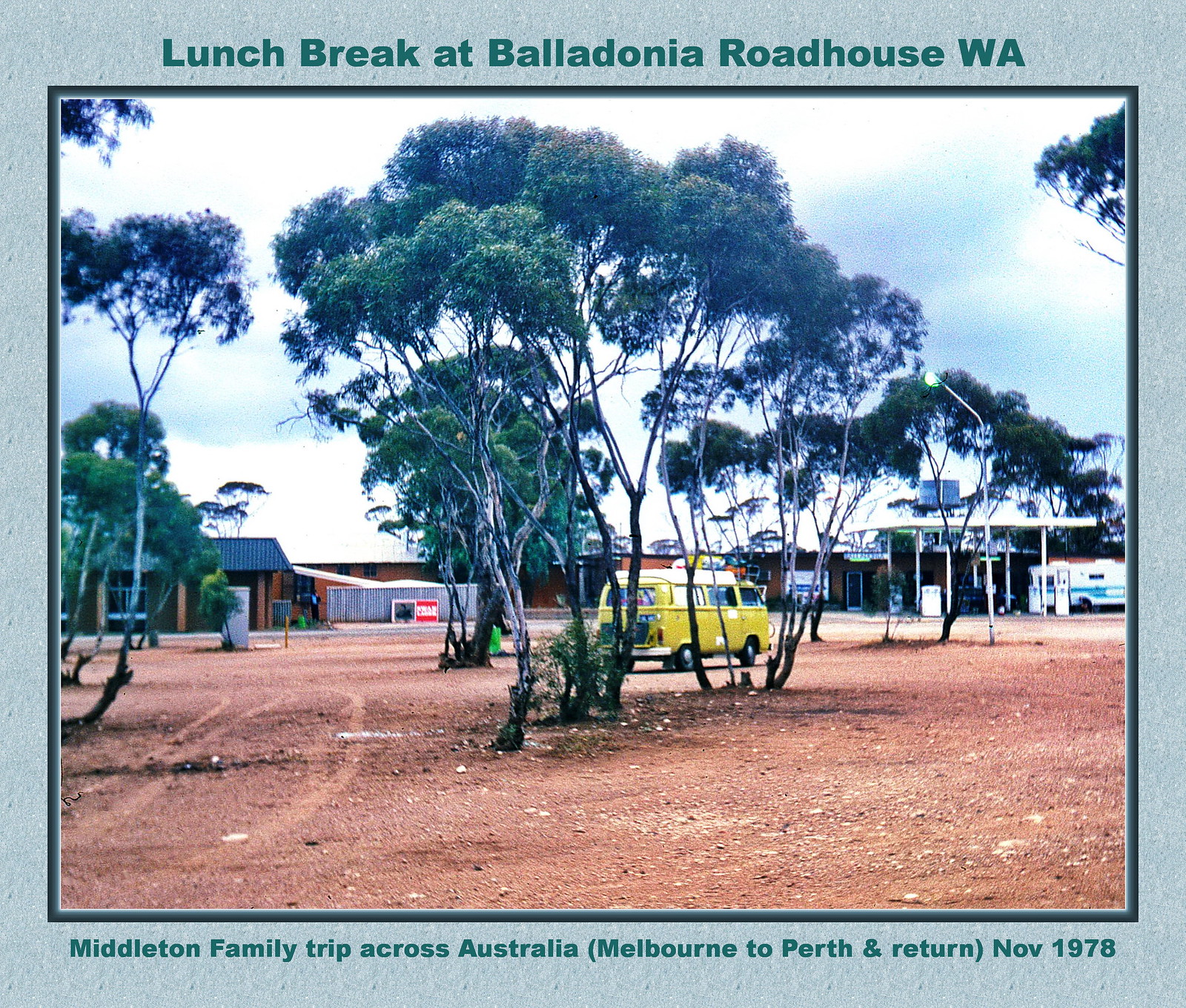This large, square photograph is bordered by a light blue frame with two lines of green text. The text at the top reads "Lunch Break at Balladonia Roadhouse, WA," and the text below the image states, "Middleton Family Trip Across Australia (Melbourne to Perth and Return), November 1978." The central image captures an outdoor setting dominated by a mostly dirt-covered ground, sporadically dotted with small rocks and narrow tree trunks bearing branches and green leaves.

In the middle ground, framed by the trees, stands an older style yellow van, evocative of the 1970s, possibly suggesting the family's mode of travel. Beyond the van, a single-story building with a black hipped roof and brown stone or brick walls is visible, alongside a smaller sheet metal building. To the right of these structures is a gas station, identifiable by its white awning supported by poles and with visible gas pumps underneath. The backdrop of the image blends into a sky filled with white and gray clouds, indicative of a typical day during their journey.